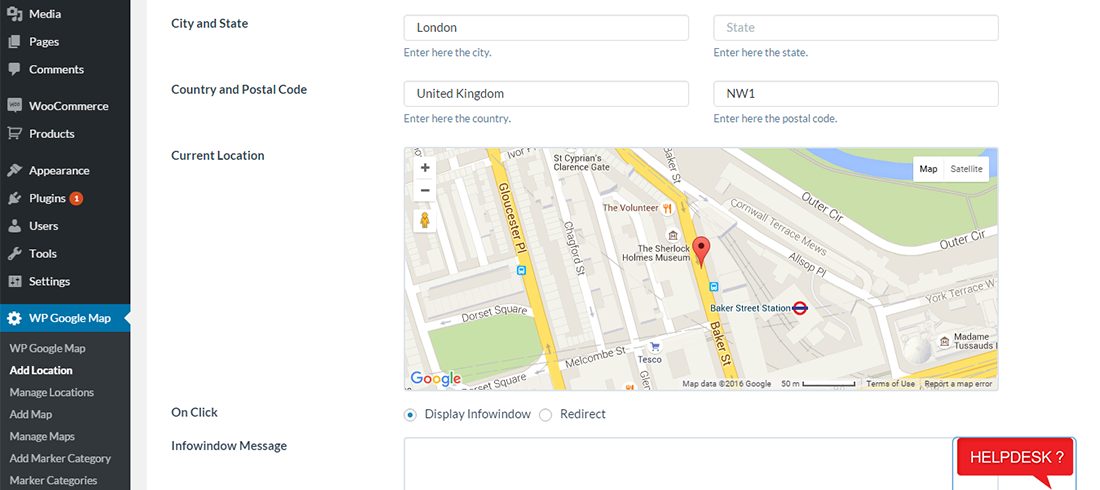**Caption:**

The screenshot displays a detailed interface of a Google Commerce management system. In the bottom right corner, there is a section labeled "Help Desk." At the very top, there are multiple tabs labeled "Media," "Pages," "Squares," and "Comments."

The central section features various dropdowns and buttons, including "Products," "Card Delay," "Appearance," "Brush Delay," "Plugins," and a large circle icon. Additionally, there is a "Persons and Users" plug icon and a wrench icon labeled "Tool Settings."

A notable blue gear icon is present, identified as "WPA Google Map." Below this, there is an option labeled "WPA Google Map, Add Location" in white, along with "Manage Locations," "Add Map," "Manage Maps," "Add Market Category," and "Market Categories."

The interface also includes fields for location data: "City and State" with "London" as an example, "State" with instructions to "Enter Here the State," and "Country and Postal Code" showcased as "United Kingdom, NW1." Further options include "Enter Here the Country" and "Enter Here the Postal Code," along with a "Current Location" feature and a visible map.

The map displays various locations and landmarks including "Glow," "Sisterville," "Baker Street," "Volunteer," "Sherlock Holmes Museum," "St. Students," "Glen Street," "Outer Circuit," "Overall Transmissions," and "LSUP." The map data is credited to Google, dated 2016.

Additionally, there is a display option for an Info Window, which is shown as unchecked, as well as a "Redirect" option and an "Info Window Message."